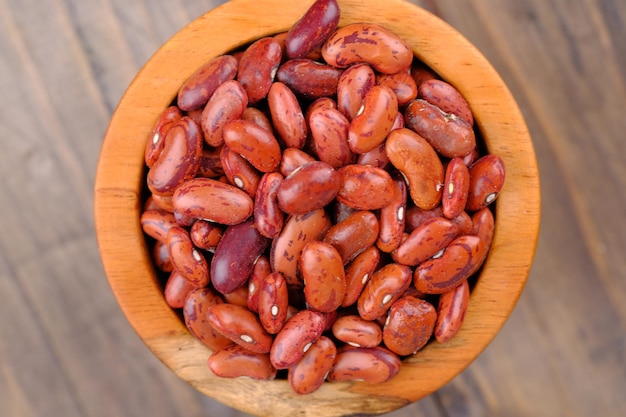This image showcases a detailed, aesthetic, top-down view of a wooden bowl filled to the brim with approximately one or two cups of dry pinto beans. The bowl, perfectly centered on a wooden table, emphasizes the rustic simplicity of the scene. The beans themselves are predominantly light brown with darker red splotches and speckles, each displaying unique patterns and textures, including small, distinct white eyes. The close-up perspective captures the intricate details and variety in color, making the beans appear almost like a cross between beans and peanuts. The overall composition highlights the natural beauty and texture of the dry beans against the blurred, wooden background.